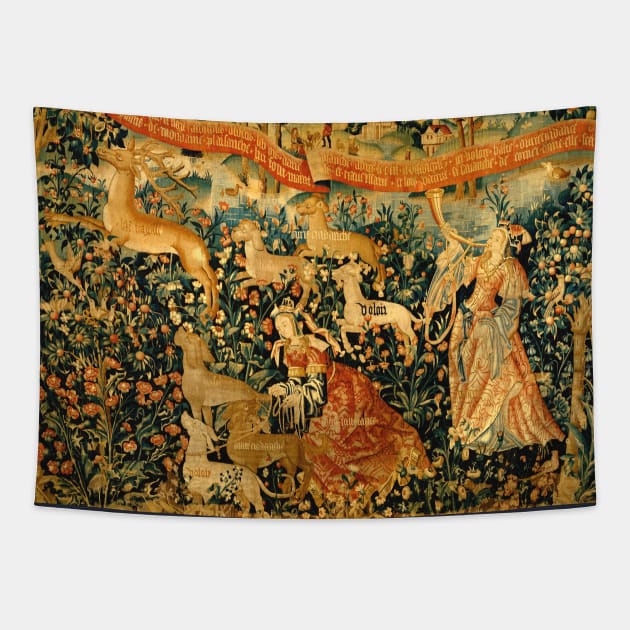This image captures a detailed, almost rectangular tapestry-like painting laid against a light grey surface that forms the background. The fabric, with its subtly curved edges, appears to have a forest-inspired scene. The foreground depicts a dense, dark green field adorned with orange and white flowers. Amidst this vibrant plant-covered ground, two women are distinctly portrayed; one is seated and dressed in a darker orange gown, interacting with a group of animals, while the other stands elegantly in an orange gown, blowing into a long, ornate horn.

The animals, depicted in various shades of brown and gold, include a mix of dogs and deer. A prominent golden-brown deer with large antlers stands to the left, accompanied by smaller, similarly colored deer. Scattered around them, there are several brown and lighter-colored dogs.

In the background, there are two orange banners with yellow writing, suggesting a narrative or message written in an unrecognizable language. These banners drape across the upper portion of the image, adding to the rich tapestry-like quality. Beyond them, a hint of a residential area with houses and trees completes the scene, creating a harmonious balance between natural beauty and subtle human presence.